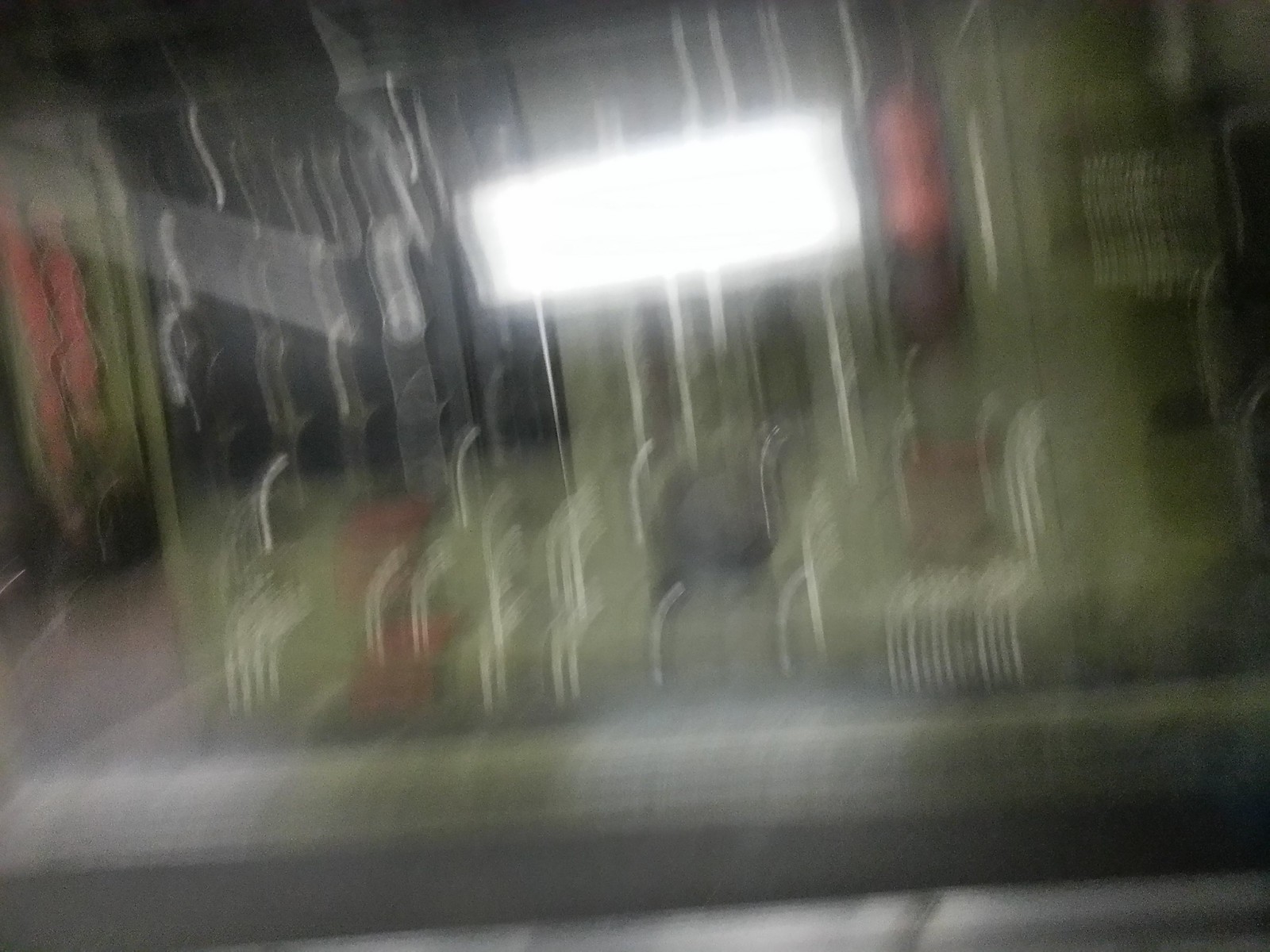This highly blurred indoor photograph depicts what appears to be a countertop cluttered with various items, including an indistinct machine. A narrow, wide band in the background could be either a window or a light source, though the heavy blurriness makes it difficult to discern. The color palette includes shades of gray, light army green, dark tones, and hints of red, all blending together in the indistinct, fuzzy composition.